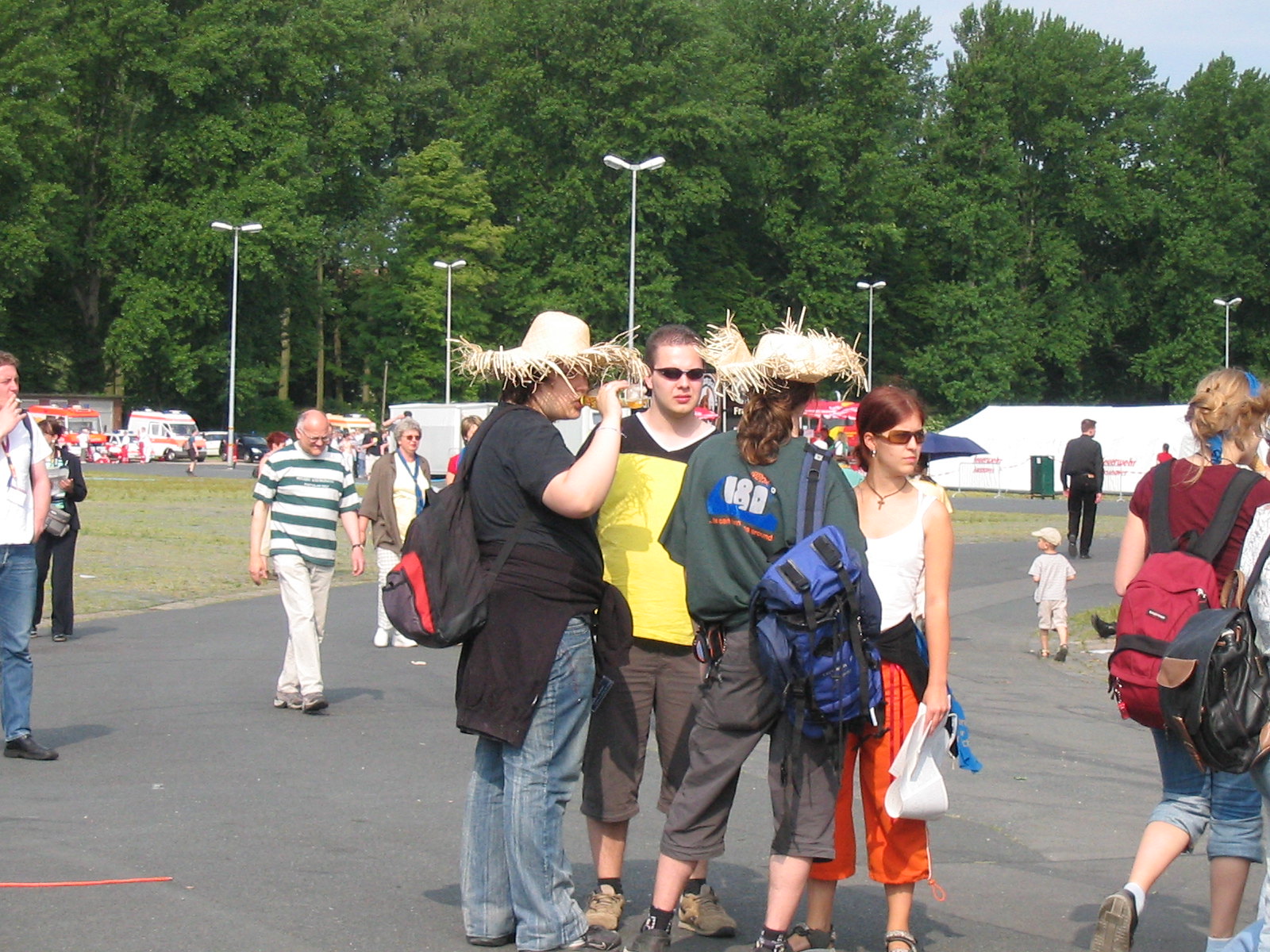In this image, a group of people is gathered outside on a sunny day, likely participating in an outdoor event or gathering. The scene is set on a paved concrete road with trees and streetlights in the background, suggesting it might be a park or a parking lot. Several children are in the foreground, with a couple wearing straw hats and milling about. There are people of varying ages, including older individuals and a child walking nearby. Some notable figures are a man in a yellow shirt, black shorts, and shoes, and a woman in a white top, orange pants, and sandals. 

Two adults wearing straw hats are central to the image; one has a black shirt and another a green shirt with "480" on the back. A lady in the foreground wears a blue backpack on one shoulder, while a man nearby has a straw hat, a black backpack, and a sweatshirt tied around his waist. Numerous attendees are seen with backpacks, and a man to the left is smoking a cigarette. Additionally, a tent with red lettering, likely for the event, is visible in the background.

Remarkably, an ambulance and several emergency vehicles like fire trucks are stationed in the background, implying a proactive safety measure for the event. The entire gathering has a laid-back, social atmosphere, enhanced by people drinking beverages and chatting casually. The image captures a blend of leisure and organization on a bright, clear day under a blue sky.